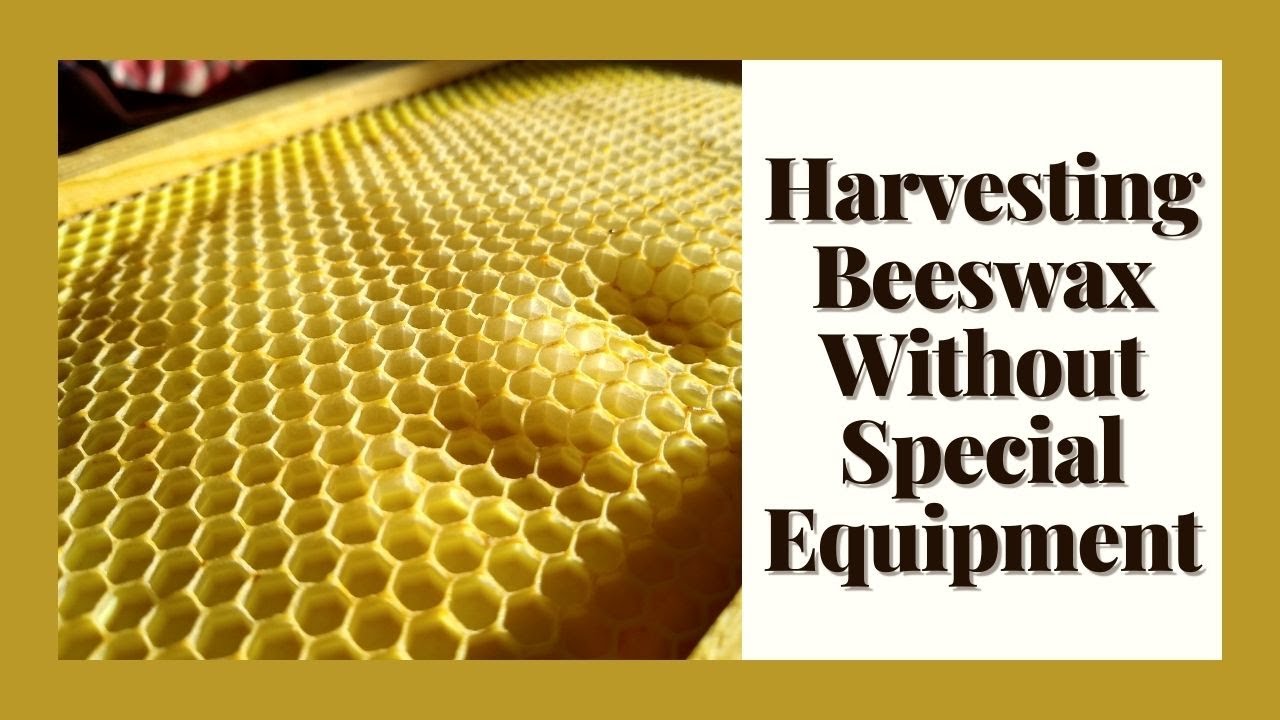The image is a rectangular, wide photograph resembling a header for an article or tutorial. It features a honeycomb encased in a light brown wooden frame on the left side. The honeycombs are golden-yellow, meticulously arranged, suggesting they are part of a controlled honey harvesting setup rather than in the wild. In the upper left corner, there is an out-of-focus red and white object, possibly a flower. Surrounding the entire image is a golden-honey colored border, adding to the thematic consistency. On the right side of the image, there is a white rectangular field with bold black serifed text that has a subtle grey drop shadow. The text reads: "Harvesting beeswax without special equipment." The image’s design blends the visual appeal of the honeycomb with informative text, effectively highlighting the subject of the tutorial or article.